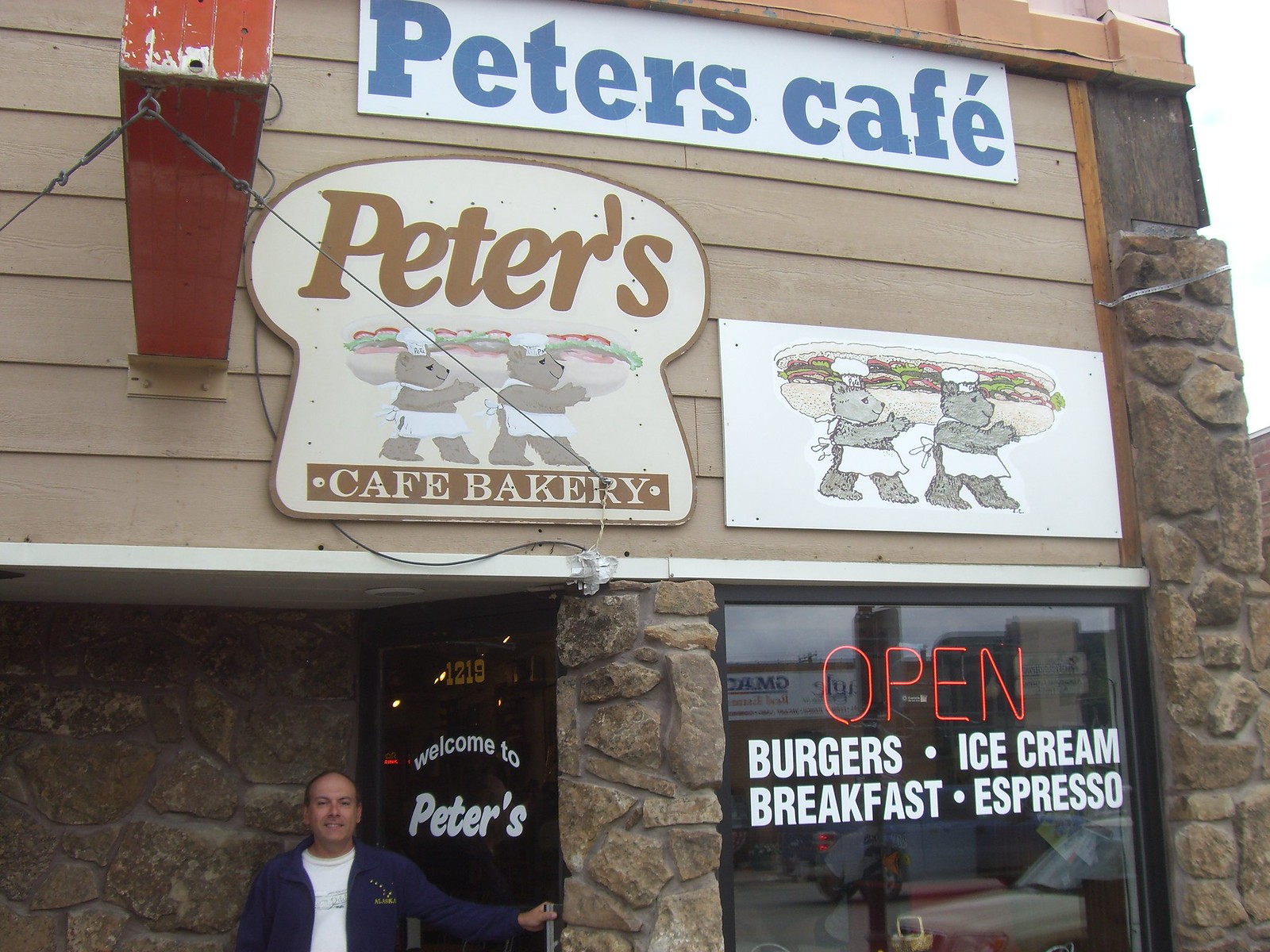The image depicts the exterior of Peter's Cafe, characterized by distinct signage and charming details. The main sign at the top reads "Peter's Cafe" in dark blue font against a white background. Beneath it, a bread-shaped placard declares "Peter's Cafe Bakery" and features two beige teddy bears dressed as bakers, complete with chef's hats and white aprons, carrying a colorful submarine sandwich filled with lettuce and tomatoes. Adjacent to this, there is another sign displaying just the bears with the sandwich.

To the left, a smiling gentleman, likely Peter, stands at the door. He wears a white t-shirt under a blue jacket and has his hand on the door handle, warmly inviting guests with a "Welcome to Peter's" sign on the glass. The building itself has beige-tan siding with stonework around the door and along the lower section of the facade. The door has the building number "1210" above it. Neon lights in the window glow with the word "Open," and the glass lists offerings such as burgers, breakfast, ice cream, and espresso. The overall setting is brightly lit by natural sunlight, enhancing the welcoming atmosphere.